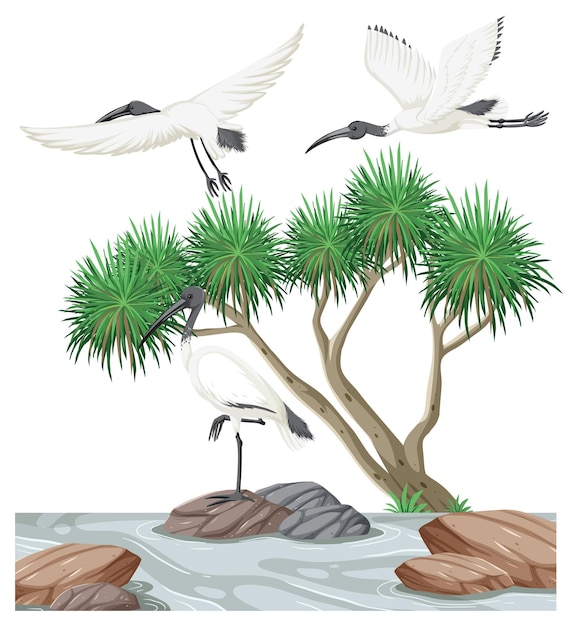This is a highly detailed digital illustration with a portrait orientation. The image features a serene scene against a white background, which likely represents the sky. Dominating the top of the image are two elegant birds, possibly storks, flying gracefully. These birds have predominantly white bodies with black-tipped wings, dark grey heads, long black beaks, and extended long legs trailing behind them.

At the bottom of the illustration, there is a tranquil water scene with several large, brown and grey rocks scattered throughout. On the central rock, a similar bird stands on one leg, while its other leg is tucked neatly beneath its body. The bird showcases its striking features, including a long black beak, a black head, and black legs.

In the background, partly submerged in the water, a distinctive tree with pointy brown stems and fuzzy, pom-pom-like green foliage adds a tropical touch to the scene. The water itself is depicted in varying shades of grey. The entire image, with its cartoon-like style, combines these elements to create a cohesive, peaceful vignette.